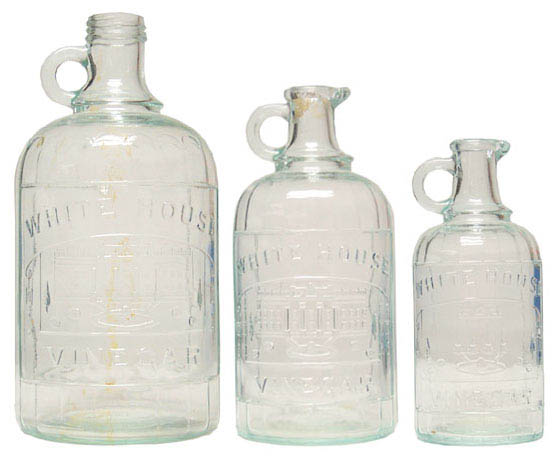The photo depicts three clear, mostly opaque jugs of varying sizes arranged from left to right against a white background. The jug on the left is the largest, the middle jug is medium-sized, and the one on the right is the smallest. Each jug features a small, half-circle handle near the top for easy holding. The handles resemble a "C" shape. The bottles appear empty, and faint text on them suggests the letters "W," "US," and possibly "White House." The writing on the bottom of the largest jug could indicate contents like vinegar, though it's not entirely clear. There is no additional context or objects present in the image.